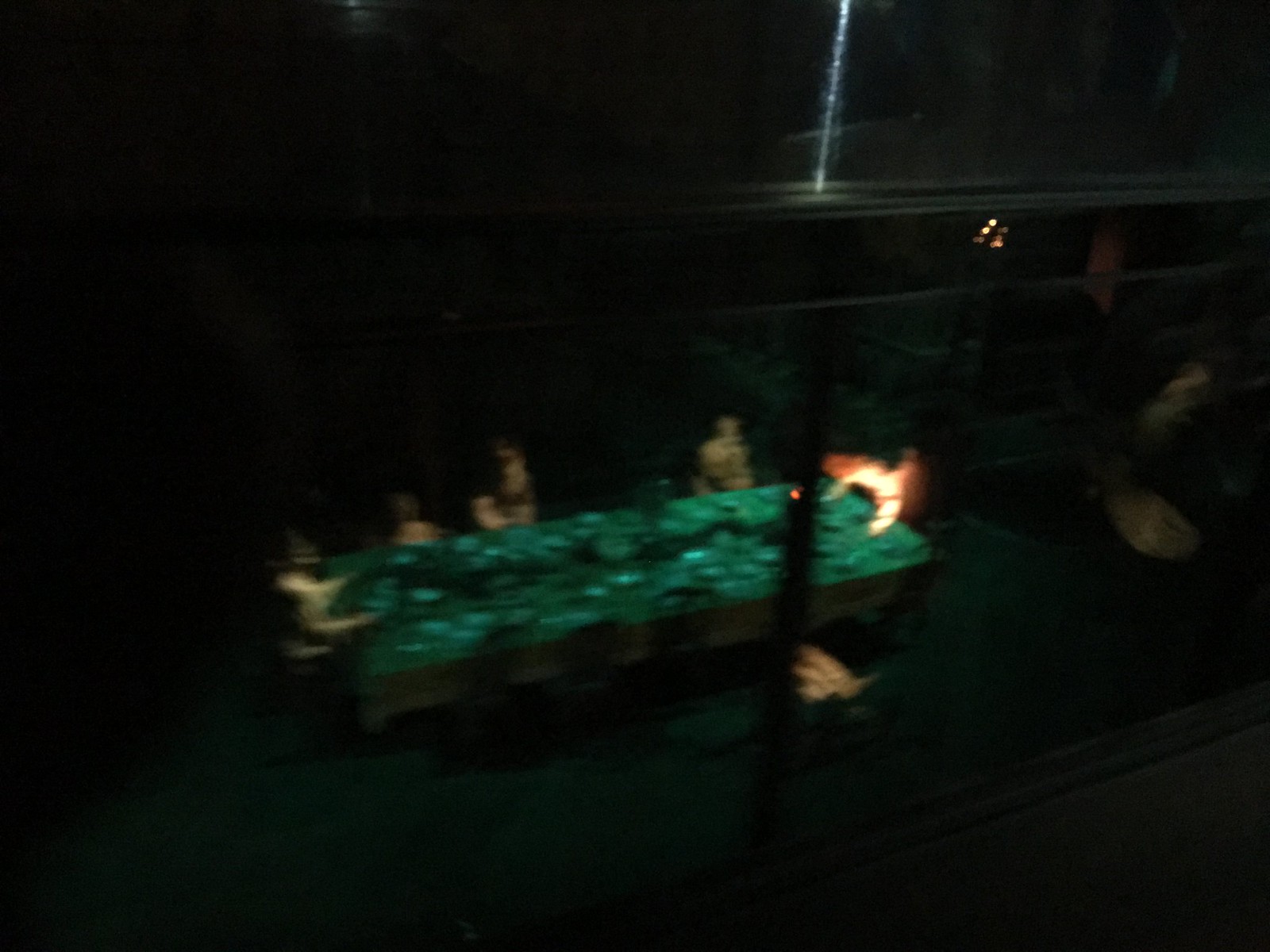This photograph-style, computer-generated image portrays a super grainy and very blurry view of people seated at a long rectangular table, viewed from above with a slightly tilted perspective. The table, featuring a green surface with lighter green circles and a black wavy line running down its center, is populated by a mixture of adults and children. You can discern taller figures and shorter ones, indicating the varied ages of the seated individuals, although their faces are indistinguishable due to the blurriness.

White or light-colored dishes are scattered across the table. The head and foot of the table each host a person, while to one side, a small person and two others are visible. On the opposite side, the backs of four black chairs can be seen. A noteworthy feature is a monster-like figure with wings at the head of the table, emitting a glowing light, adding an element of surrealism that blends with the reflective quality of the image.

Additionally, a white line descends from the top right of center and touches a black horizontal rectangle, from which a black pole extends downward, further contributing to the chaotic and mysterious atmosphere of the scene.